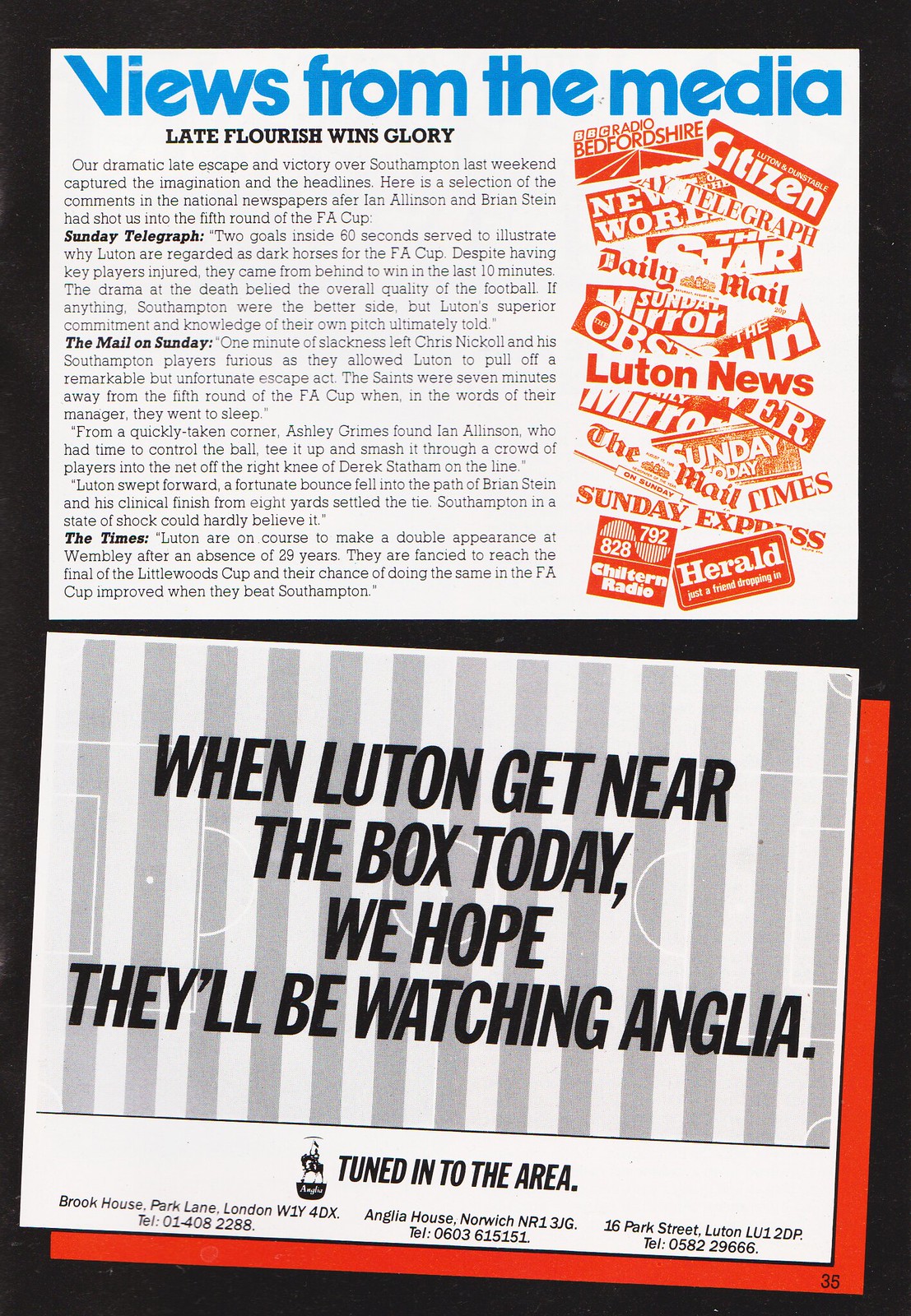The image appears to be a page from a magazine or newspaper featuring two distinct sections, one above the other. The top section, titled "Views from the Media" in blue text on a white and gray background, showcases comments and reviews from various newspapers about a game, specifically highlighting "late flourish wins glory." Beside this heading, logos of prominent newspapers such as the Sunday Telegraph, the Mail on Sunday, and the Times are displayed, created in orange, red, and white colors, and they appear as if they were cut and pasted. The lower section is an advertisement with a red background layered with gray and white stripes. It reads, "When Luton get near the box today, we hope they'll be watching Anglia," and includes tuning information for the area. This ad also bears some addresses and telephone numbers, indicating it is London-centric.